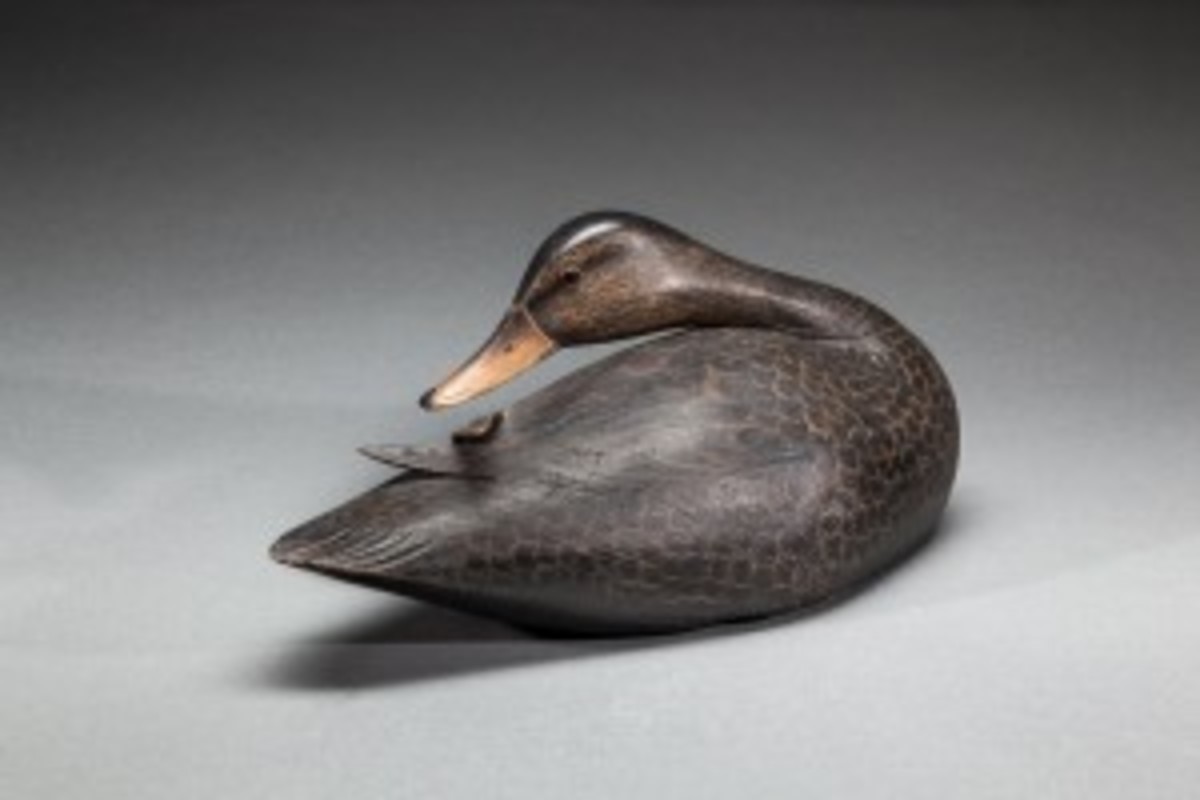The photograph captures a wooden duck statue set against a seamless gray backdrop with a gradient effect, darker in the upper corners and lighter near the bottom. The highly detailed carving depicts a mottled, dark brown and black duck with a glossy finish, reflecting light off its body and head. The duck’s intricately carved feathers, particularly notable at the rear where they appear to stick up, offer a textured, lifelike detail. Its head is turned backwards to the left, as if looking over its body, bringing attention to its realistic, glossy black eyes and a light orange-gold beak with black accents at the tip and base. The statue mimics a resting or swimming position, evoking a natural and serene posture.